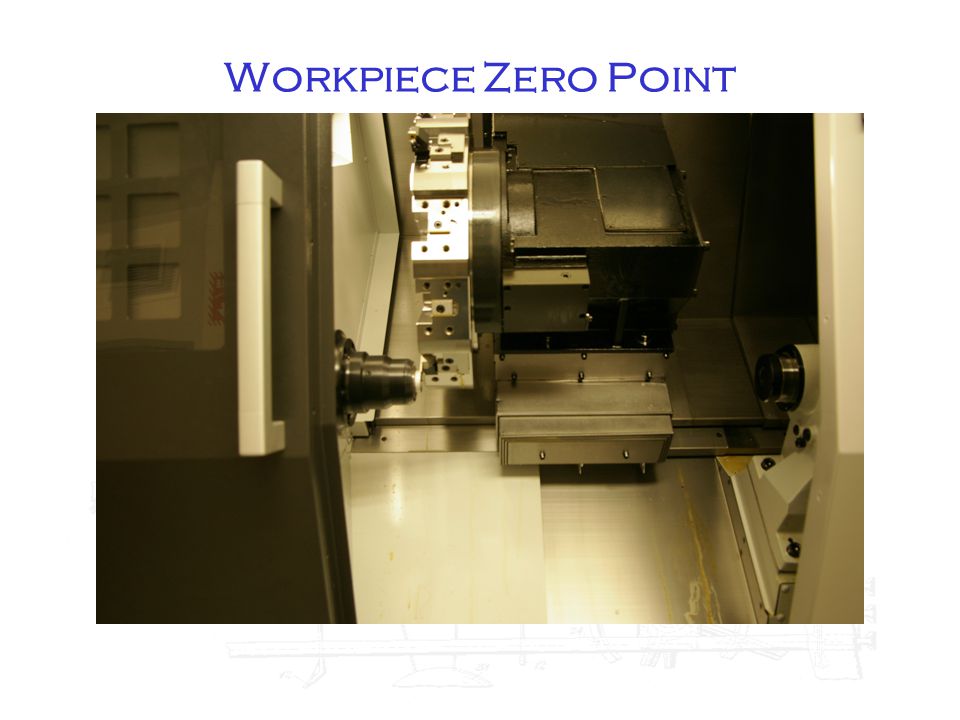The image captures an industrial indoor setting that resembles a laboratory environment. Dominated by metallic and plastic components, the photograph prominently features a complex machine with various parts, including gears, bolts, and screws. The top of the image displays the text "WORKPIECE ZERO POINT" in blue, capitalized letters against a white background. On the left side, a black door with a grid-like pattern and a silver handle can be seen. The equipment itself, positioned mainly in the center and extending to the left, includes rectangular prisms flanked by lenses, all having a metallic and shiny appearance. The surface textures range from smooth, off-white walls resembling those found in clinical settings, to reflective, gray metallic surfaces. The photograph provides a detailed glimpse into a specialized, high-precision industrial environment, replete with intricate machinery and orderly arrangement, captured under good lighting conditions that highlight the shine of the metal parts.